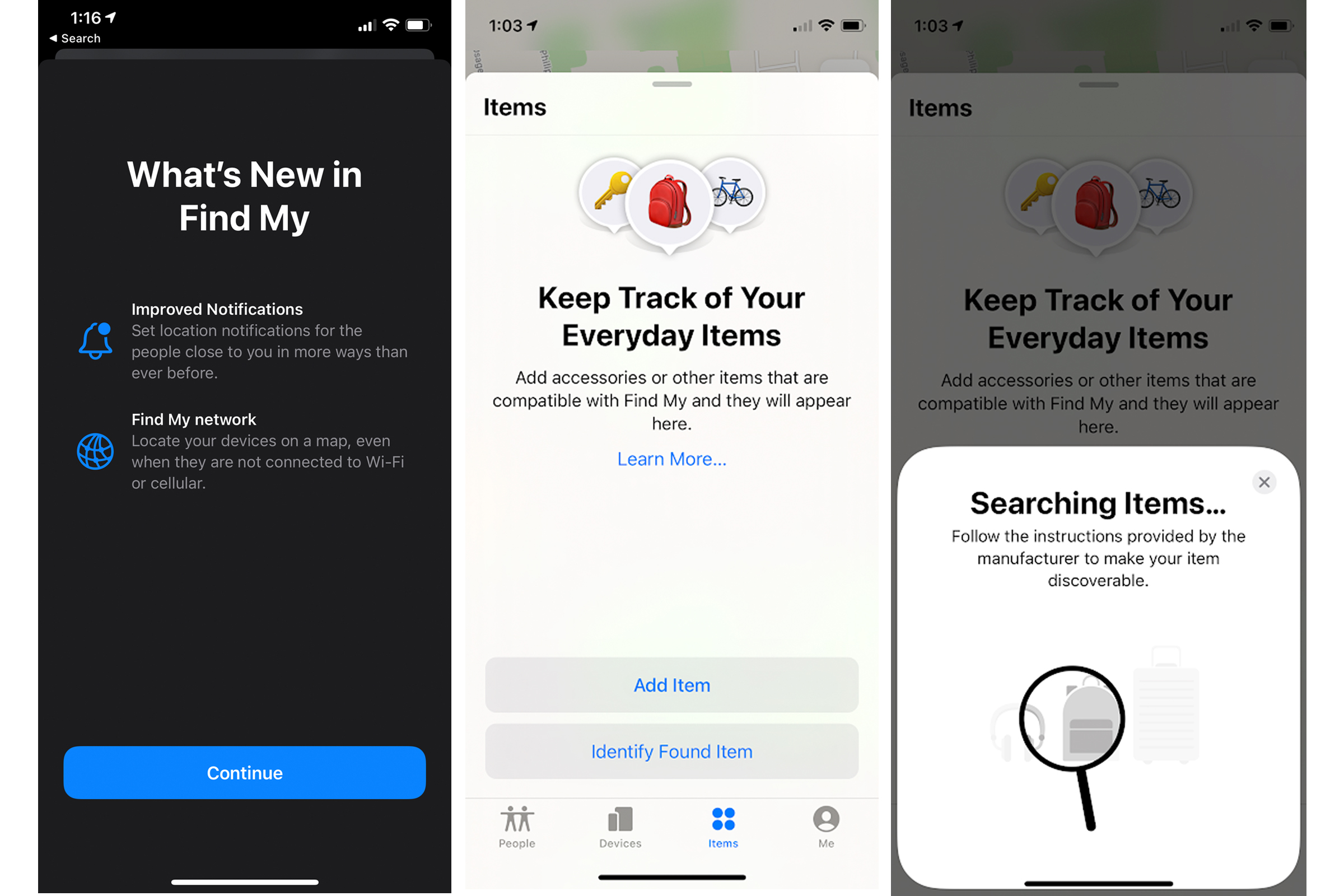The image showcases three different screenshots from an iPhone, all displaying various functionalities of the "Find My" app. 

The first screenshot (on the left) highlights the newest features of the app. It includes a detailed explanation about enhanced notifications and the capability to locate devices on the map even when they are not connected to Wi-Fi or cellular networks. This suggests improvements in device tracking precision and more consistent updates on device locations.

The middle and right screenshots focus on the app's core functionality. Both screenshots feature a menu with three distinct icons representing tracked items: a yellow key, a red backpack, and a blue bike. The middle screenshot illustrates the main menu, which encourages users to "Keep track of your everyday items." 

The right screenshot adds an extra layer of detail, showing a submenu that provides further options or information about the selected items. This submenu appears as an overlay at the bottom of the screen, indicating additional interactive features to manage the tracked items more effectively.

In conclusion, these screenshots collectively depict the user interface and functionalities of the "Find My" app on an iPhone, emphasizing its utility in tracking personal items and staying updated with the latest enhancements in location services.